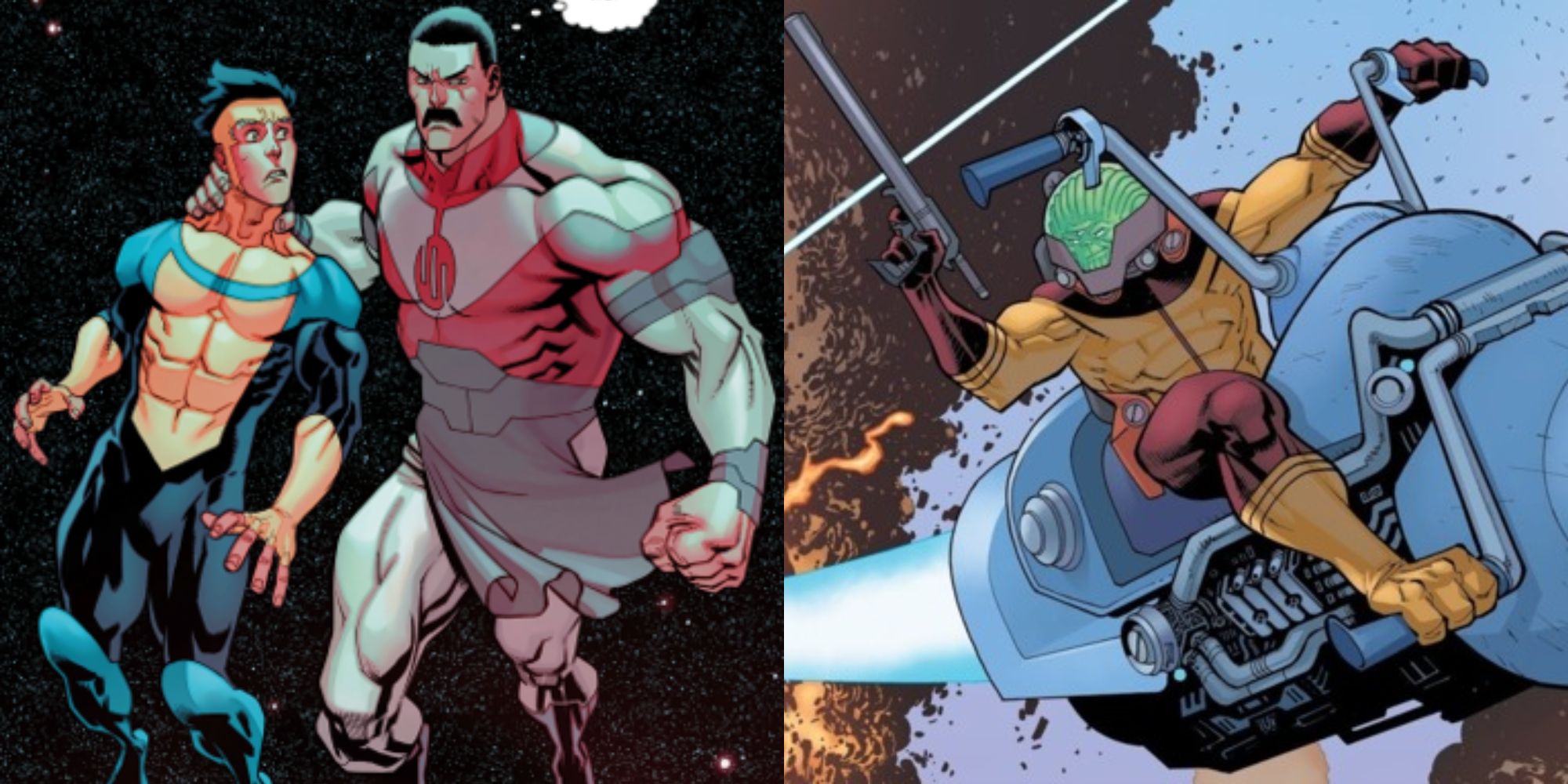In this composite image from the comic "Invincible," we observe two distinct scenes. On the left, Mark, also known as Invincible, is depicted in his blue and yellow superhero costume, standing beside his imposing father, Omni-Man. Omni-Man, characterized by his red, white, and gray attire, as well as his prominent mustache and dark short hair, is gripping Mark by the back of his neck, conveying a sense of dominance and anger. His other hand is clenched into a fist, further emphasizing his fury. They appear to be floating in space, as suggested by the surrounding cosmic backdrop. Mark looks visibly terrified in contrast to his father's menacing demeanor. On the right side of the image, an alien character, referred to by some as Mordok from the Marvel Universe, is riding a light blue space motorcycle with tall handles. This creature, with a foot resembling a palm gripping the motorcycle’s foot pegs, wields a long gun in its right hand. The alien's appearance draws a striking parallel to the character Mordok, known for his oversized head in earlier comic renditions, albeit depicted differently here.